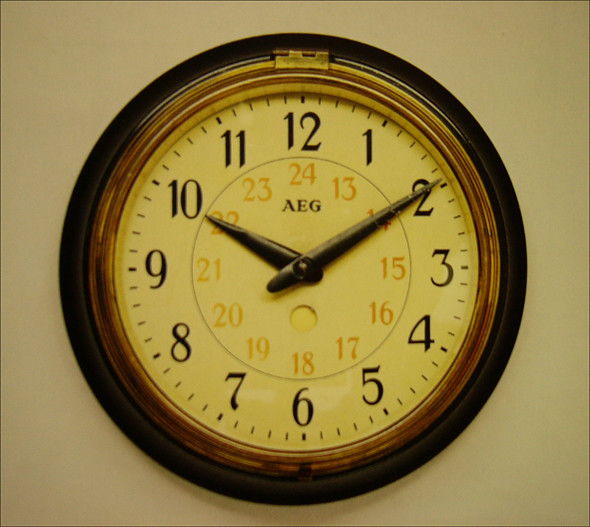This image depicts a clock set against a light brown background. The clock features a dark brown outer rim, complemented by a lighter brown border inside it. The clock's face is a light yellowish-beige color, with dark brown numbers from 1 to 12 marking the hours. Between each number, there are dark brown minute markers. The clock has black hour and minute hands. 

In the center of the clock face, there is a dark gray circle containing numbers from 14 to 24, suggesting a 24-hour format. Below these numbers, the brand name "AEG" is written in brown.